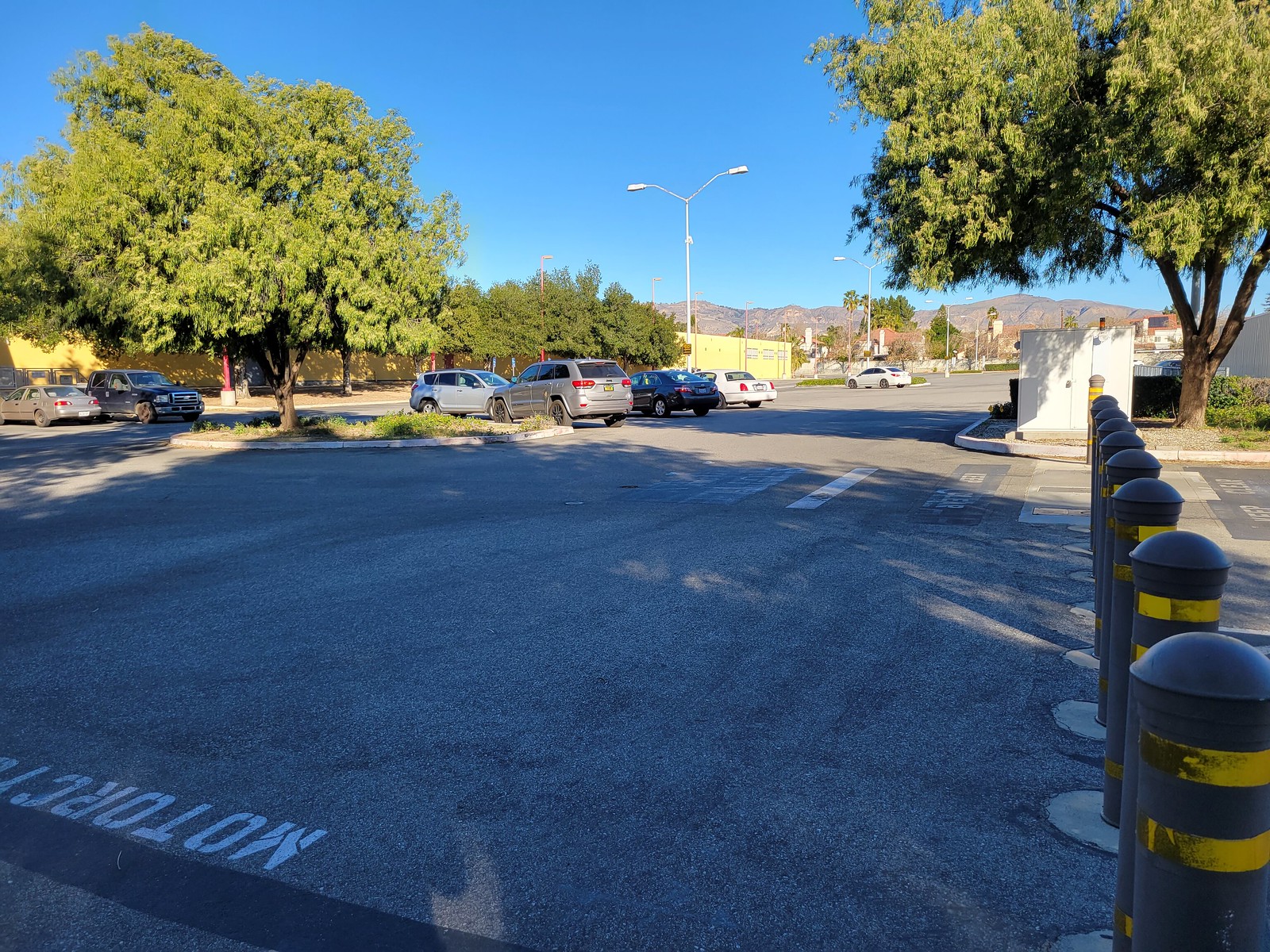The photograph depicts a moderately occupied parking lot, seemingly located in an American town, possibly in Arizona or a similar western state. Starting from the lower right-hand corner of the image, a row of approximately nine retractable hydraulic bollards is visible, strategically placed to block one lane of traffic. These bollards can be raised or lowered as needed.

In the parking area, which is shaded by a number of acacia trees, several cars are parked but the lot is not full, indicating a relatively small parking capacity. To the left, a sidewalk lined with more trees further contributes to the shaded environment. The scene suggests this is a well-maintained area, often bustling with activity.

In the background, bare high-desert mountains loom, characteristic of the region's arid landscape, with no tree line on them. Intermingled with the acacia trees are scattered palm trees, adding a distinctive touch to the otherwise sparse mountainous backdrop.

In the foreground, stenciled road traffic indicators are painted on the pavement, although they show significant wear. One such marking, partially visible, seems to spell out "MOTORCYCLE" but is cut off at the 'Y.' Additionally, faded white crosswalks crisscross the pavement, again showing signs of wear.

The far edge of the parking lot is bordered by the wall of a building or a barrier, painted in a pale yellow hue. Above this, terracotta-tiled rooftops of distant buildings contrast beautifully with the natural scenery. Streetlights and parking lot lights are strategically placed throughout the area, ensuring visibility and safety after dark.

Overall, the photograph captures a serene yet functional parking area amidst a quintessential American southwestern town.